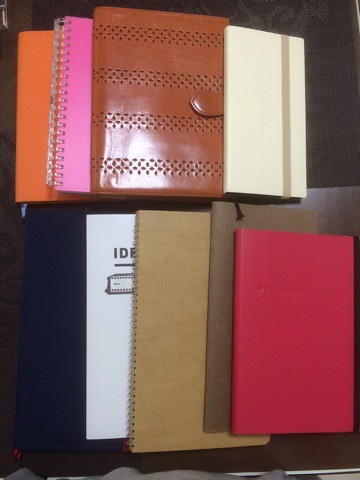The image is a detailed photograph showcasing multiple small notebooks and day planners, displayed on a brown table. The arrangement is in two rows, slightly overlapping. In the top row, at the forefront, there's a brown notebook secured with a buckle, identified by its shiny leather or plastic cover. To its left lies a pink, spiral-bound notebook, partially visible. Further left is an orange notebook, with a bookmark ribbon protruding from the bottom. To the right of the buckled notebook is another partially seen notebook with a white cover, held together by an elastic band.

The bottom row features a variety of notebooks with distinct characteristics. Central to this row is a brown notebook, with a small white piece of paper behind it that includes a diagram. Just beneath this, a notebook with a raw cardboard cover and spiral binding is discernible. There's also a blue-toned notebook, and another with visible writing hinting at "IDE" or "Ideas." Completing the arrangement is a red-bound journal, distinctly visible atop the others. The entire collection of notebooks rests against a black backdrop, creating a vivid contrast.